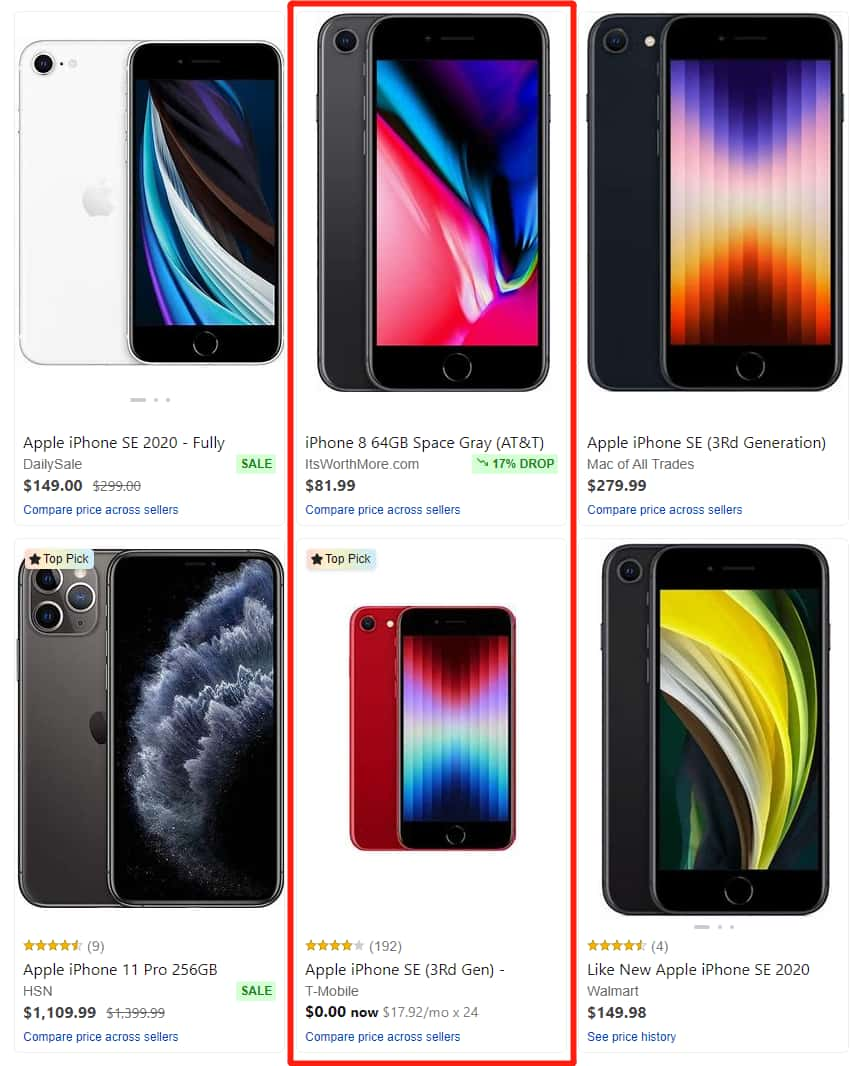This image showcases a screenshot of an online marketplace displaying six different cell phones arranged in a grid format—either two rows of three phones each or three columns of two phones each. Each phone is annotated with its model and price. 

Starting from the top left and moving clockwise:
1. The first phone in the top left corner is an Apple iPhone SE 2020 featuring a white back and a black screen surround, priced at $149.
2. Directly below it, in the bottom left corner, is an Apple iPhone 11 Pro with a black back, listed for $1,199.
3. The top center phone, encased within a large red rectangle, is an Apple iPhone 8 with 64GB storage in space gray, available through AT&T for $81.99.
4. Beneath it, also within the red rectangle, is a red-backed Apple iPhone SE 3rd generation, which is noted as "zero new," implying it is only available second hand. The price for this is unspecified.
5. In the top right corner is another Apple iPhone SE 3rd generation, this time with a black back, priced at $279.99.
6. Finally, in the bottom right corner, is a like-new Apple iPhone SE 2020 with a black back, available for $149.99 from Walmart.

The diverse range of models and conditions displayed provides a clear overview of different options and price points available for Apple iPhones on this online platform.